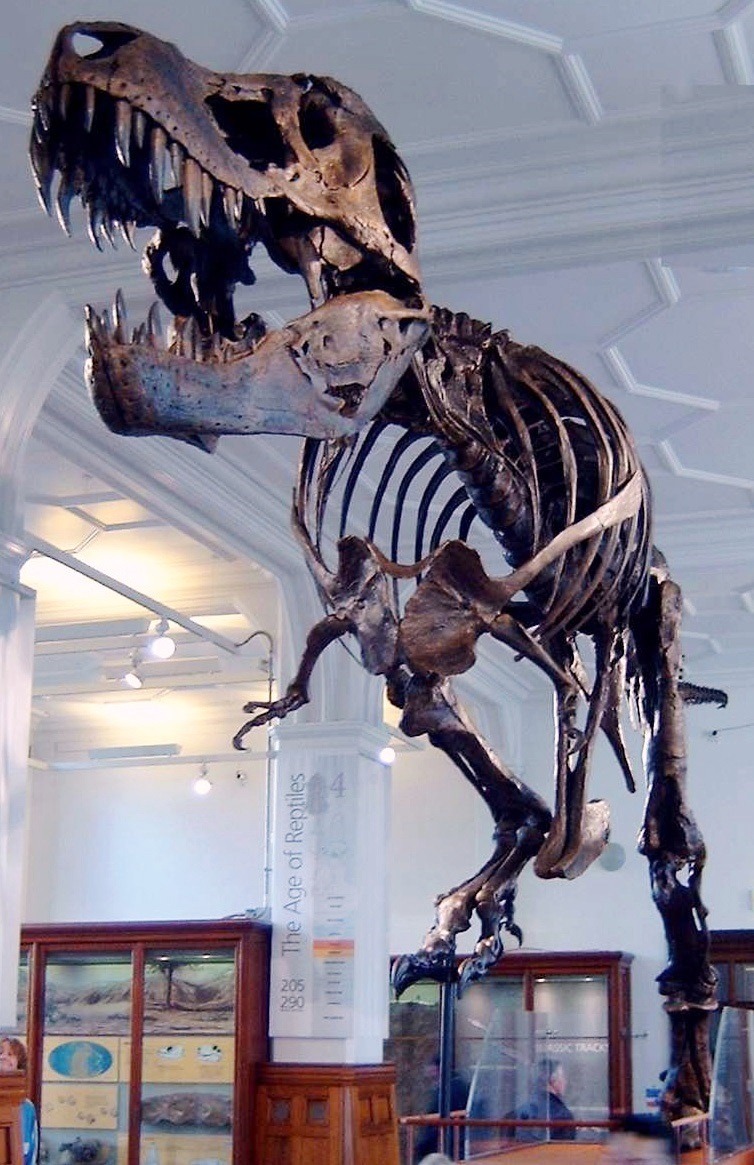The image is a high-quality photograph taken inside a natural history museum. Dominating the scene is a large, dark brown skeleton of a Tyrannosaurus Rex, mounted on discreet black metal supports. The T-Rex's mouth is open, showcasing its intimidating large teeth, and it is facing slightly to the left of the viewer. The background features warm-colored wooden display cabinets with glass fronts, containing various exhibit items. The room itself is quite spacious, with white walls and ceiling adorned with art deco patterns. Illuminated by white lights, a prominent pillar stands in the center of the room, partially brown at the base. The pillar bears the text "The Age of Reptiles" along with some numerical information and additional, smaller text that is unreadable. The photograph blurs the background slightly to emphasize the grandeur and details of the T-Rex skeleton.